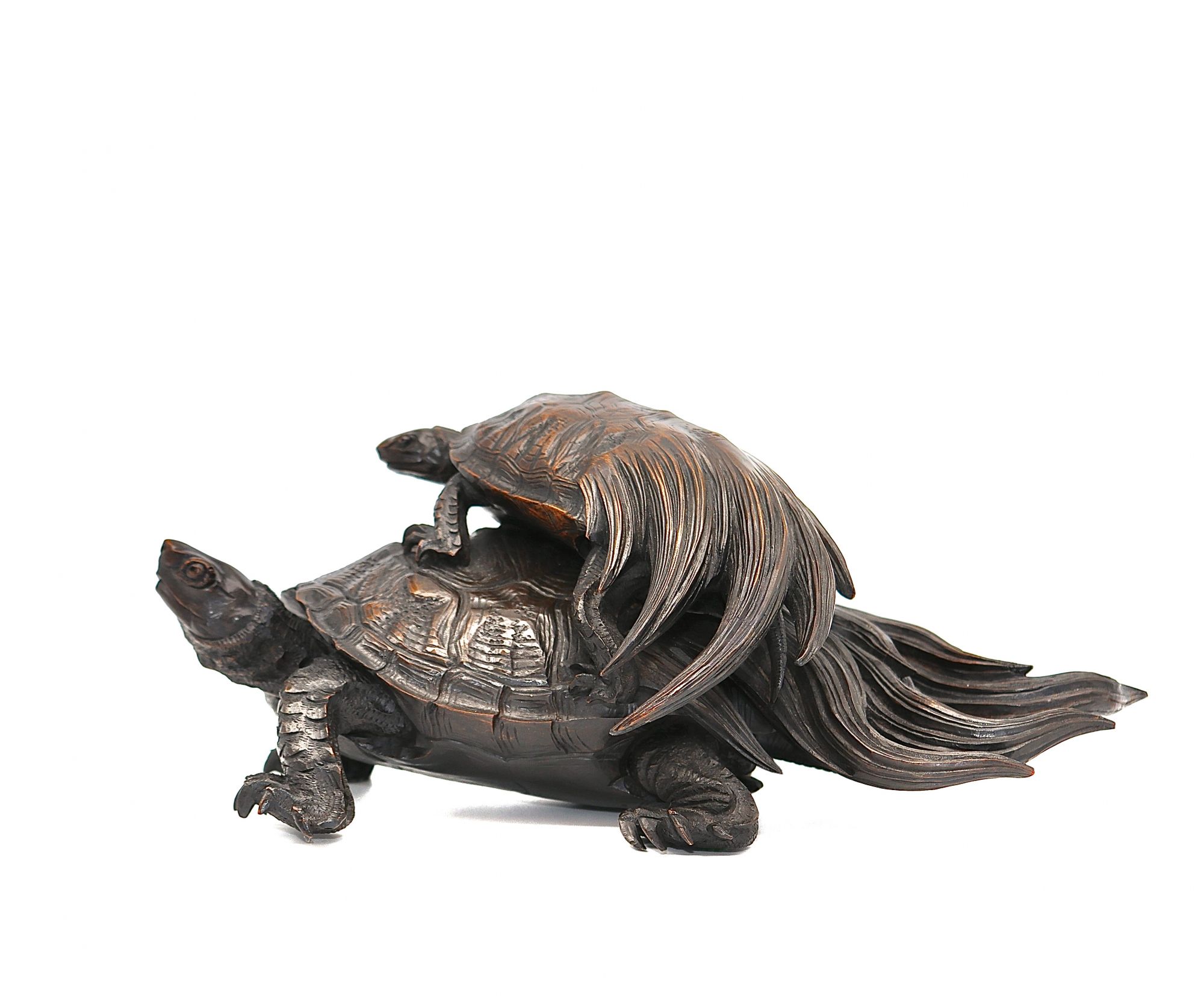The image showcases an intricate ornamental bronze statue depicting two terrapins, one larger and one smaller. The larger terrapin is positioned side-on to the camera, with its head turned to the left and raised at a 45-degree angle towards the ceiling, showcasing its detailed scale work and claws. Its shell features subtle bronze highlights and distinct patterns, while its extravagant tail curves downward like flowing peacock feathers or kelp, extending towards the ground. Perched on the larger terrapin's back is a smaller terrapin with an identical design. This smaller figure is placed at an angle, with its face turned diagonally away from the camera, allowing a clear view of its striking, flared tail pointing to the right. The smaller terrapin's shell has additional rose-gold bronzing highlights. The background of the image is entirely white, accentuating the detailed craftsmanship and unique metallic finish of the statue.